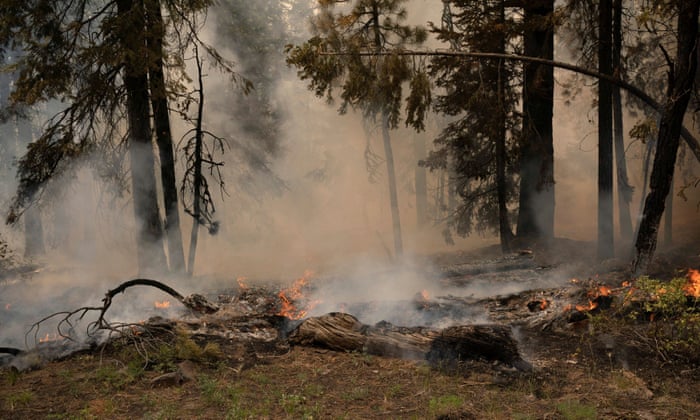In this dark and starkly contrasted image of a forest area, the aftermath of a forest fire is clearly visible. Black silhouettes of trees stretch across the background, their trunks and leaves illuminated by sporadic, small fires dotting the forest floor. A thin layer of white smoke pervades the scene, rising from what seems to be a burning dead log or branches scattered across the brown dirt. Despite the destruction, patches of green shrubs and grass survive in the foreground. Among the charred remains, one particular tree bends downward, its branches broken and damaged, possibly a pine tree. The scene is heavily smoked, with trunks especially to the left appearing badly charred and burnt foliage adding to the sense of devastation.